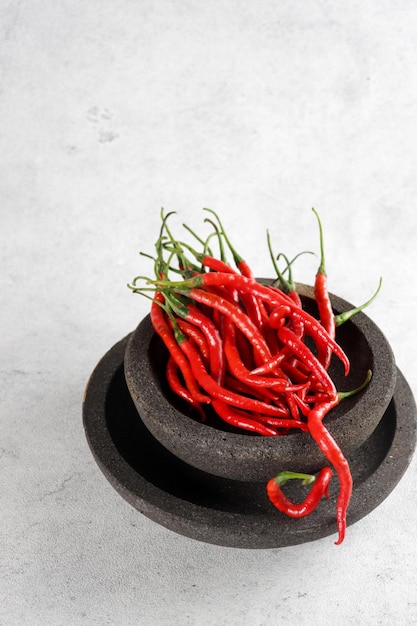The image features a collection of long, thin red peppers with green stems, arranged inside a circular, dark brown stone bowl that resembles a mortar typically used for grinding. This smaller bowl is placed atop a larger, matching stone plate of the same color and rough texture, evocative of asphalt. Both the bowl and plate are placed on a white surface with subtle gray marbling. Approximately 15 to 20 red chilies are clustered within the bowl, with a couple of them having fallen out and resting near the lower right-hand side of the plate. The entire arrangement sits prominently on what resembles a chalky, grayish-white concrete surface.